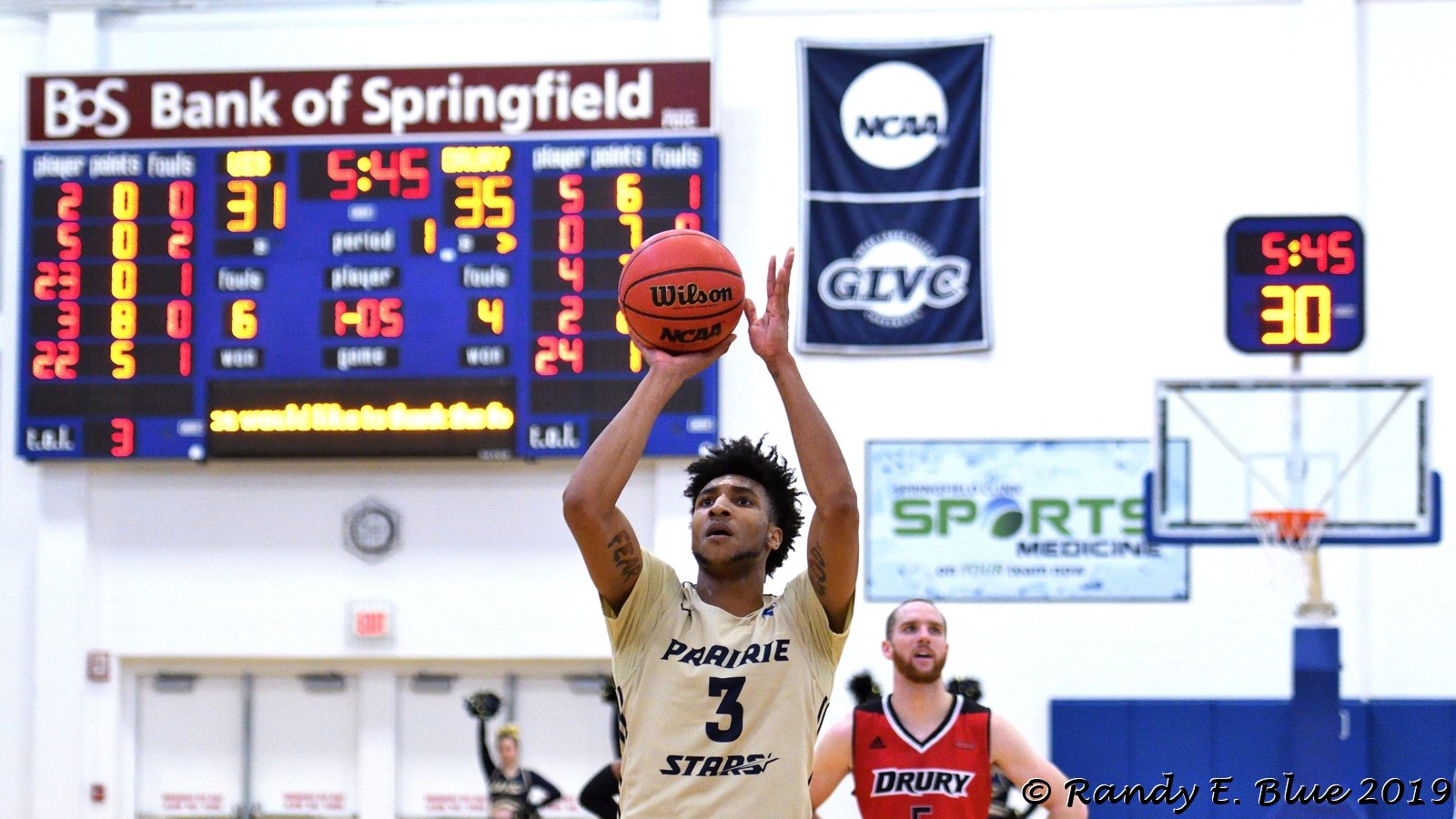This detailed photograph captures a dynamic moment in a college basketball game between the Prairie Stars and Drury. Central to the image is a young black player from the Prairie Stars, wearing a yellow jersey with black text, number three, captured mid-motion as he prepares to shoot a free throw. In the background, a white player from Drury, identifiable by his full beard and red jersey with black text, stands ready. The setting is an indoor arena, visually anchored by a scoreboard located in the upper-left corner that reads "Bank of Springfield" with a score of 31 to 35, indicating 5 minutes and 45 seconds left in the first period. The scoreboard emits a mix of blue, yellow, and red lights and presents various game statistics. Adjacent to the scoreboard, the shot clock aligns with the time display. The background features a white-walled arena adorned with NCAA and GLVC signs, and cheerleaders in black uniforms holding black pom-poms stand near emergency exit doors, enhancing the vibrant atmosphere of the game.